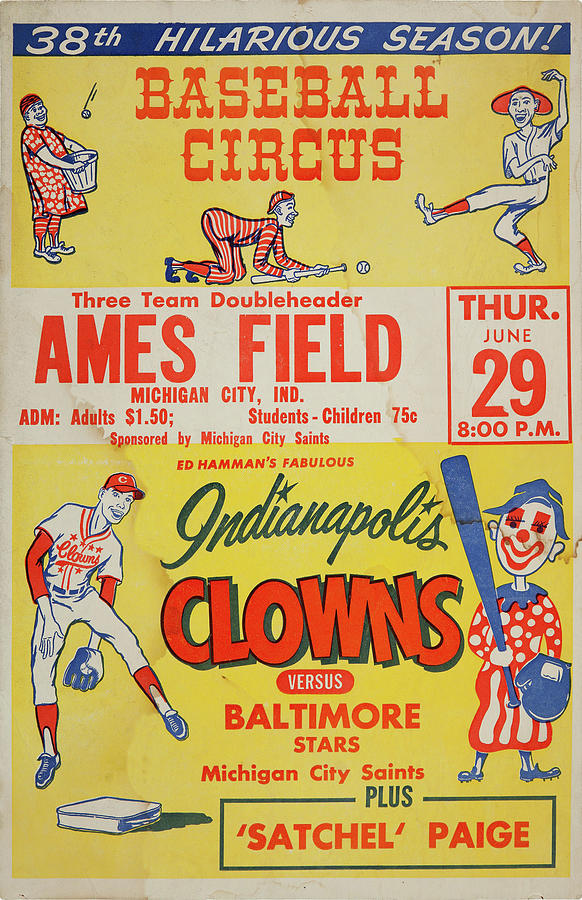The poster, which seems very old and weathered, features a bright yellow background with a white border around the edges. At the top, within a blue rectangular strip, bold white text announces the "38th Hilarious Season." 

Below that, in large red letters, it reads "Baseball Circus." The center of the poster is filled with lively, animated illustrations of clowns and baseball players in humorous scenarios: one clown in a long red robe with spots and striped pants is catching a ball in a bucket, another character is crawling on the ground using the wrong end of a bat, and a third character, wearing a long-brimmed hat, is dancing.

In red and white text, the event is detailed as a "Three Team Doubleheader" taking place at "Ames Field, Michigan City, Indiana." Admission prices are listed as "$1.50 for adults" and "75¢ for students and children." The event is scheduled for "Thursday, June 29th at 8 PM" and is sponsored by the "Michigan City Saints." The bottom of the poster announces the teams and special guests in blue and red text: the "Indianapolis Clowns," "Baltimore Stars," "Michigan City Saints," plus the legendary "Satchel Paige."

Accompanying the text are additional illustrations: on the left, a baseball player, and on the right, a clown holding a baseball bat and glove, reinforcing the whimsical theme of the Baseball Circus.